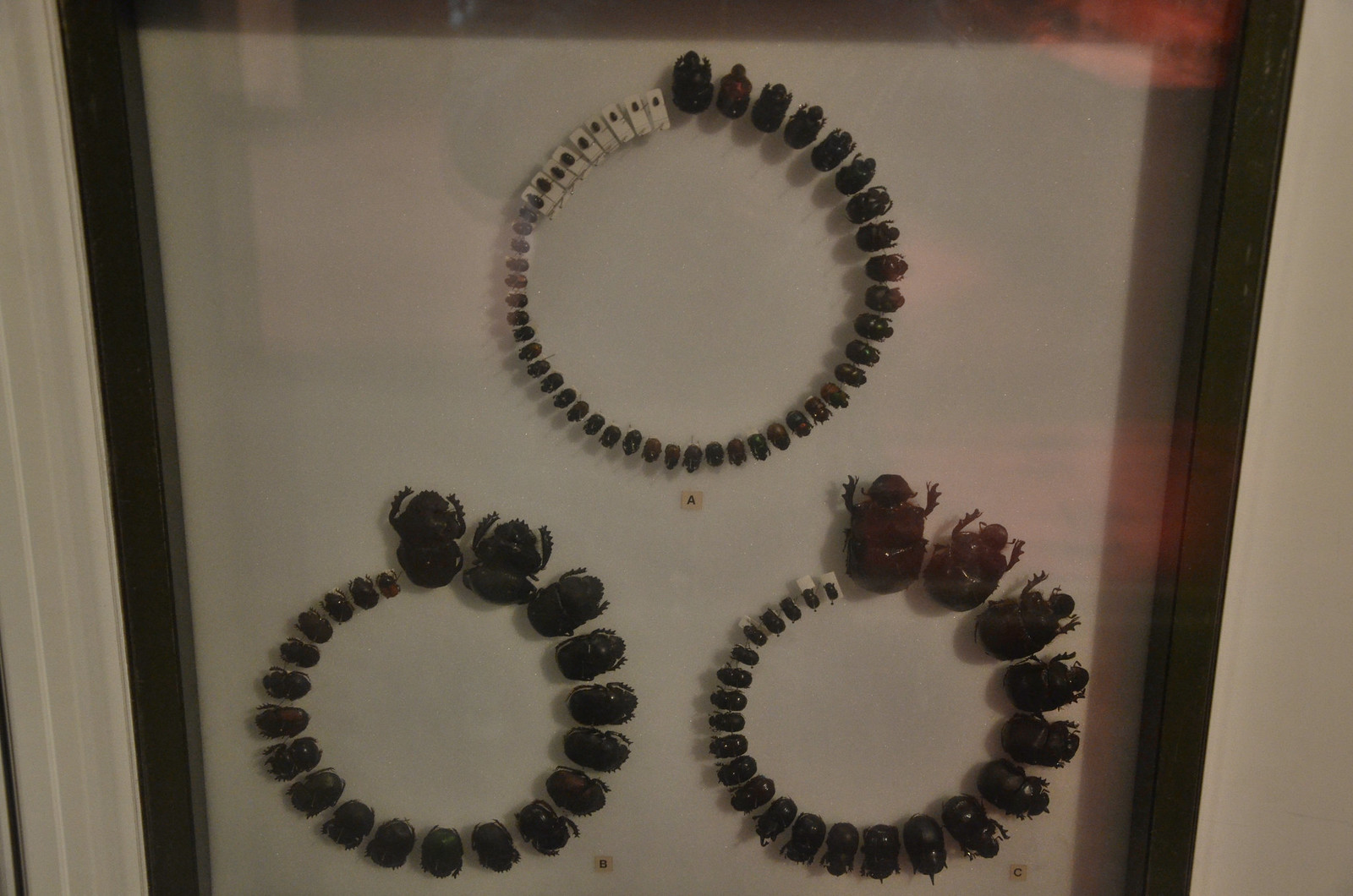The image showcases a framed display of three bracelets, each crafted from beads arranged to illustrate the growth cycle of beetles, encased behind a glass with a black inner border and a white frame visible at the edges. At the top center lies bracelet A, featuring smaller, rectangular white beads that increase in size through numerous stages, forming a petite beetle at its apex. Below, bracelet B on the lower left and bracelet C on the lower right share a similar design but with significantly larger beads, clearly defining the beetles at their peak stages. The beads on these lower bracelets are predominantly black; however, bracelet C may exhibit a brownish hue or a shadow, distinguishing it slightly from bracelet B. The display is labeled with A, B, and C in black, indicating each bracelet's position and sequence. Additionally, the glass case captures a reddish reflection in the top right corner, adding a subtle color contrast to the composition.